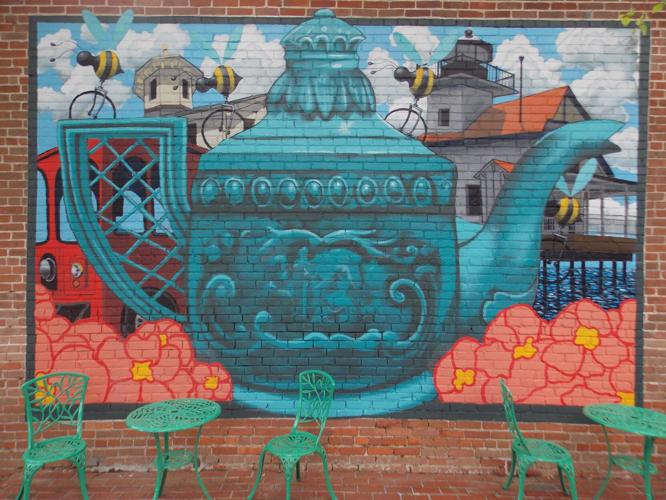The image depicts a detailed mural on a brick wall featuring a massive turquoise teapot with intricate designs, including a curved pattern in the center and oval-shaped patterns near the lid. The teapot's handle, resembling a gate or fence texture, is positioned on the left, while the opening is on the right. The mural incorporates additional artistic elements such as red and yellow flowers at the base, a blue sky with clouds at the top, and bees scattered throughout. In the foreground, there are actual green metal circular tables with matching chairs; on the left, one table is accompanied by two chairs, while on the right, a similar table has one chair to its left. The scene suggests the setting of an outdoor cafe. Behind the teapot within the mural, there appears to be a pier extending into the water and a building, integrating the mural seamlessly with its surroundings.